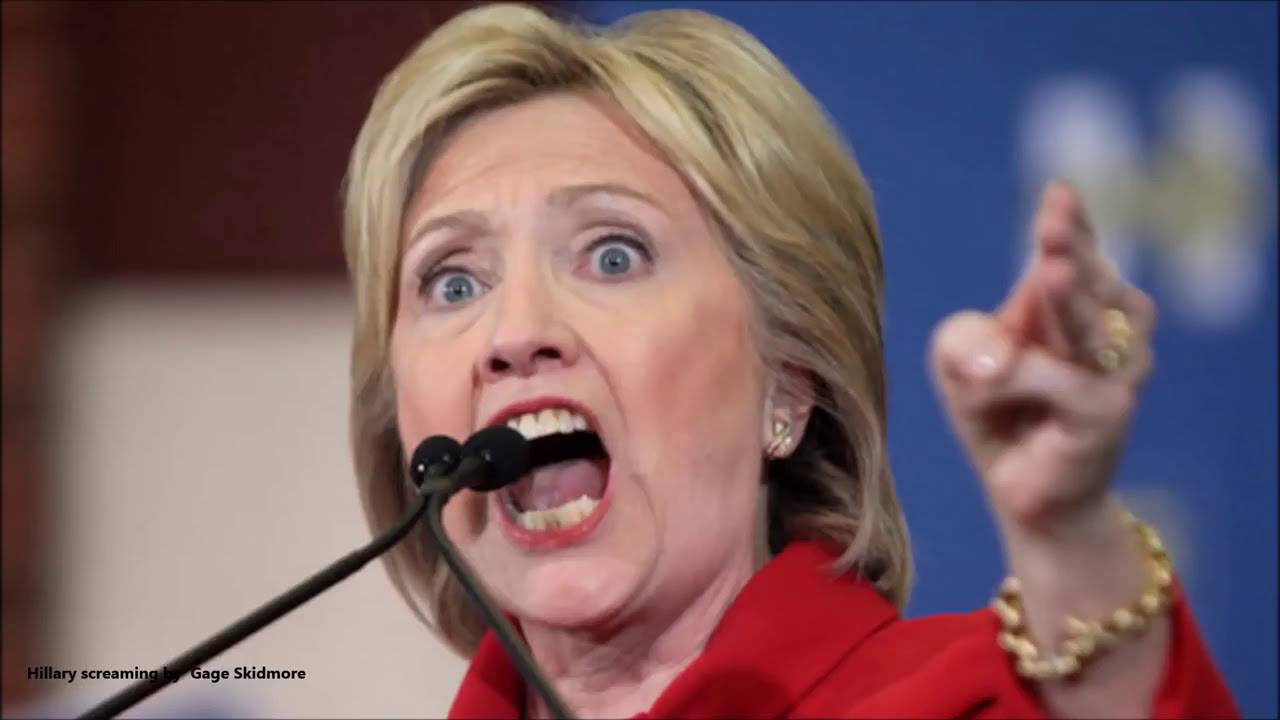The image features Hillary Clinton in mid-speech, her mouth wide open, revealing both her top and bottom teeth and her tongue. She is speaking into a black microphone with dual points at the end, held close to her mouth. Clinton's eyes are wide open, showing their light blue color, and her blonde hair, parted slightly to the side, cascades down to her neck, concealing her ears. She wears a vibrant red blazer, accentuated by a gold-colored bracelet and ring. Her left arm is lifted and extended outward, though it appears out of focus, with her thumb and pinky finger held together, pointing with the remaining three fingers. The background is blurred with shades of blue, brown, and tan, and features white logos. At the bottom left of the image, text reads "Hillary screaming" by Gage Skidmore.